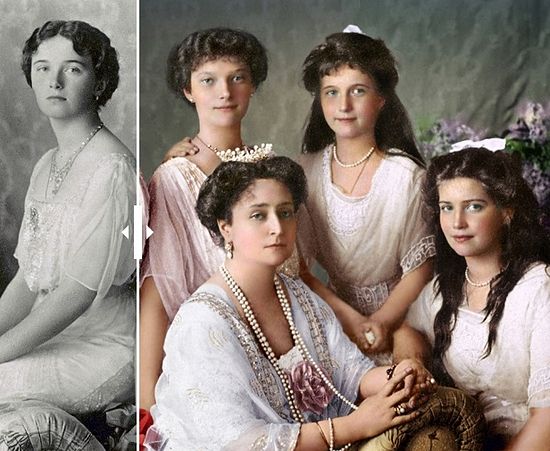This photograph depicts a group of five women seated and posing with neutral expressions in what appears to be a turn-of-the-century portrait. The image is divided into a black-and-white section on the left and a colorized section on the right. The woman on the far left, depicted solely in black and white, has short hair, a white gown, and multiple necklaces and earrings.

In the colorized section, four women are dressed in white or off-white dresses with varying hairstyles. The central figure, presumably the mother, wears a tiara, diamond earrings, and a double strand of pearls. She is flanked by a woman with a white dress adorned with floral patterns around the sleeves, wearing a white pearl necklace, and a taller woman in a pinkish dress with short hair and also adorned with a necklace. The youngest girl, positioned on the far right, has long black hair with a white bow, vibrant blue eyes, and red lips, matching the lipstick of her companions. Above her head, lilac flowers add a touch of color to the otherwise gray background.

Each woman, whether in black and white or color, is detailed meticulously, portraying a cohesive family unit despite the different hues and tones.